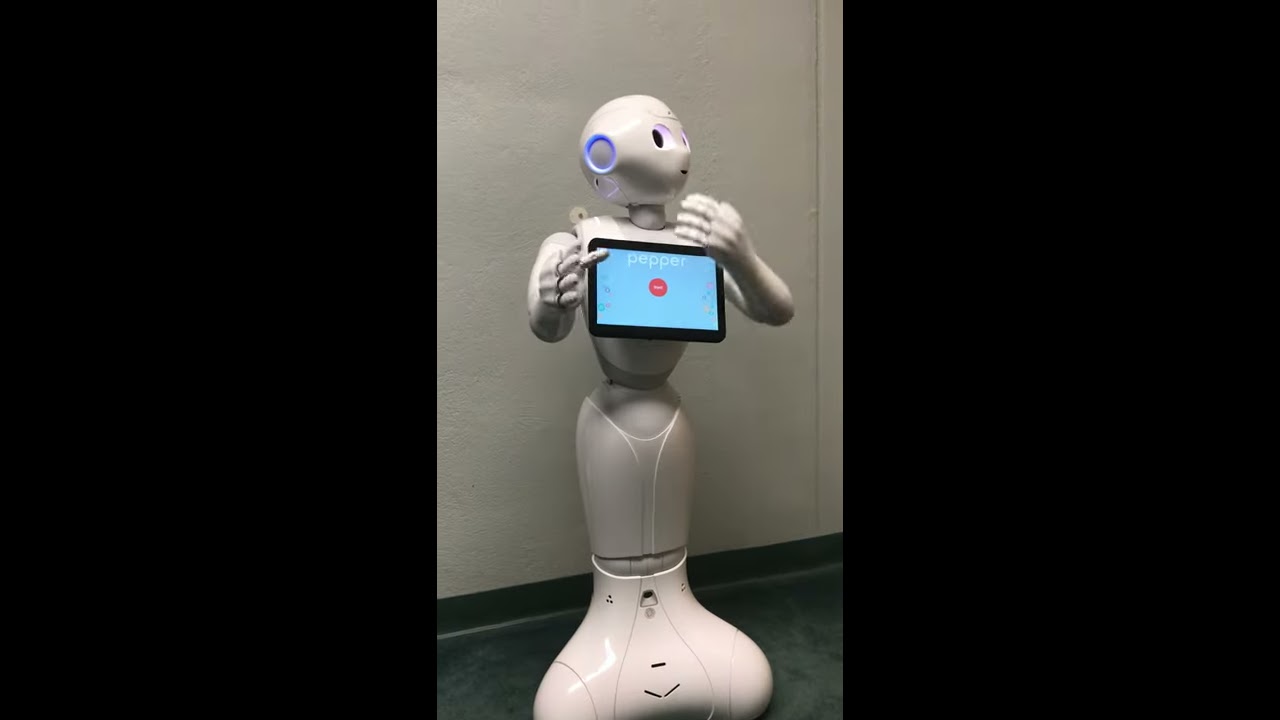The image depicts an indoor scene with a central focus on a humanoid robot named Pepper. The photograph is framed by blacked-out sections on the left and right thirds, creating a border effect around the central, taller-than-wide rectangular picture. Pepper, the robot, is positioned against a white wall with a green baseboard and green floor. 

The robot features an off-white color and stands on a base that flares out like a fishtail, suggesting a mermaid-style lower half, without distinct feet. Pepper's head is rounded and slightly turned to the right, displaying a simplistic, cartoonish face with basic human-like features including circular eyes and a small mouth. A blue circle represents the ear. 

Pepper's body faces forward and holds an iPad in its right hand. The tablet has a black outline and a light blue screen with the word "Pepper" displayed in white lettering, accompanied by a prominent red button. The iPad's exact icons and additional text are somewhat indistinct due to the distance of the camera. The overall setting appears to be a hallway or similar indoor environment, with the robot likely in motion or at least capable of movement, indicated by various joints in its structure.